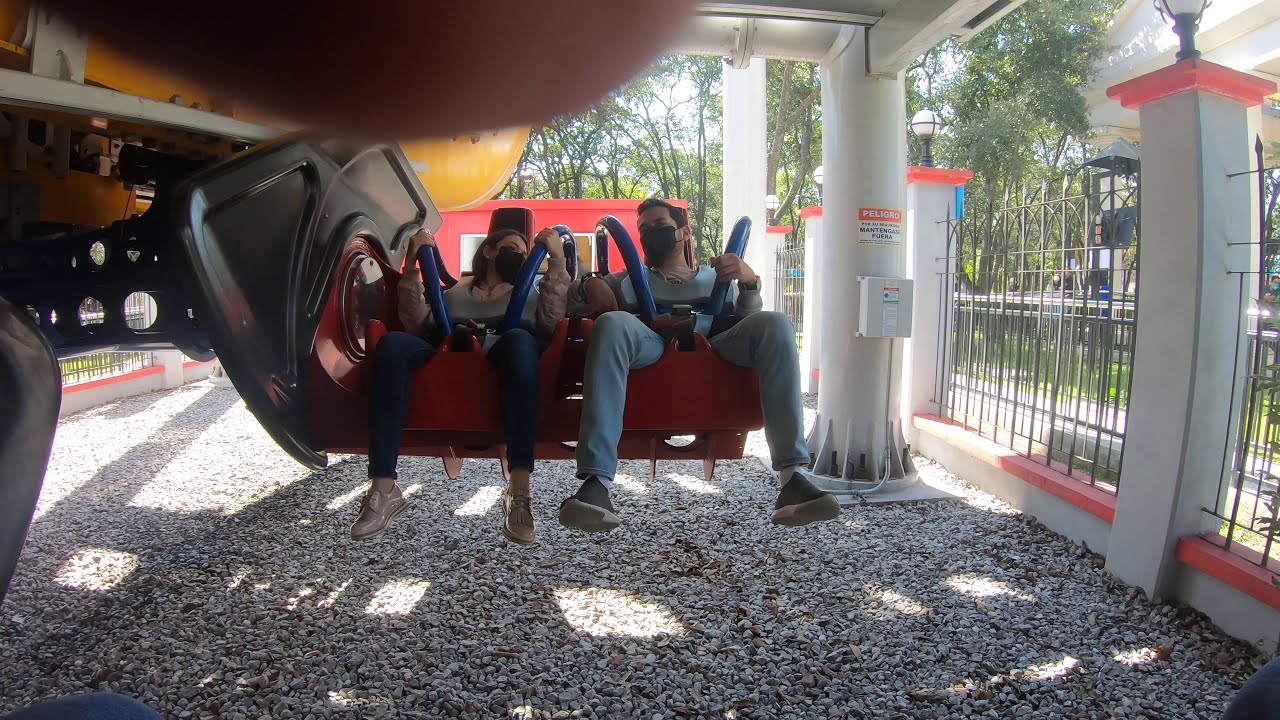In this detailed image, a man and a woman are prominently seated in the center of an amusement park ride, which takes place outdoors on a gravel surface. Both adults are clad in light tops, jeans, and colorful sneakers, and they are wearing black face masks covering their noses and mouths. The ride features a red container with a tall black wing on the left side and blue safety bars arching over and securing the riders. White columns and a black metal fence are visible on the right side of the image, along with some trees and buildings in the background. A sign with Spanish writing on one of the pillars suggests that this amusement park might be in a Spanish-speaking country. The image is taken during the daytime and a finger has accidentally been captured in the photograph. The color palette includes tan, yellow, white, black, gray, red, green, blue, and yellow.